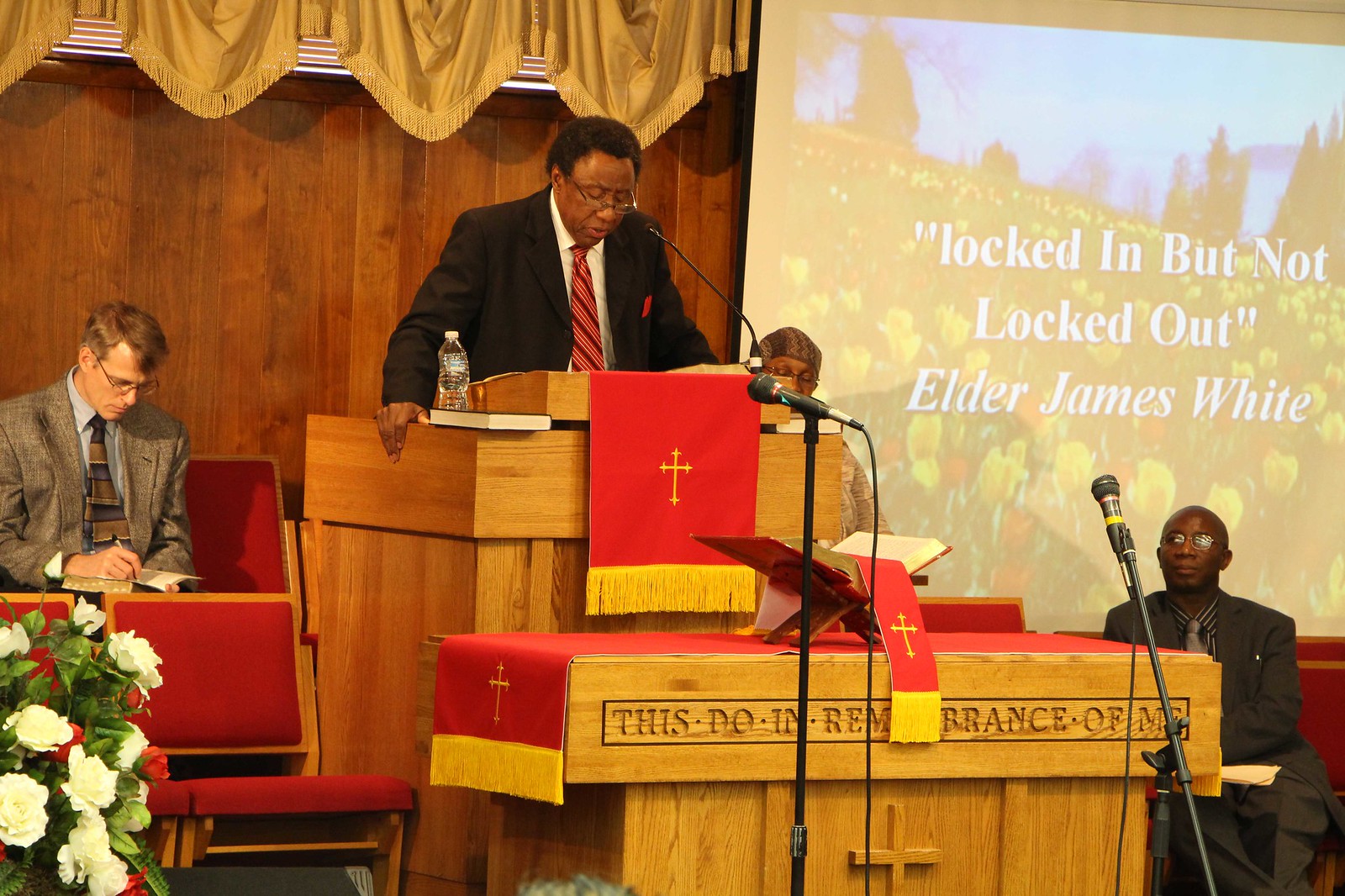The photograph depicts a detailed and reverent scene of a religious service within a church. At the forefront, an African-American gentleman stands at the wooden pulpit, dressed in a dark suit, white shirt, and red tie, with eyeglasses accentuating his focused expression as he addresses the congregation. The pulpit is draped with a red banner that features a gold cross in the center and yellow tassels along the bottom. On the light pine altar beneath him, inscribed with "Do this in remembrance of me," rests an open prayer book similarly adorned with a red drape.

Two microphones on stands flank the speaker, who extends his arms to the sides of the pulpit, creating an image of engagement and passion as he delivers his sermon. Surrounding him, other gentlemen in suits are either standing or seated on the wooden chairs, absorbed in following the service with Bibles in their laps.

A colorful projection screen to the right depicts a serene field of flowers with the text "Locked in but not locked out, Elder James White," suggesting the theme of the sermon. This scene is accentuated by the gentle presence of white flowers on the altar, enhancing the sense of solemnity and devotion. The image captures the moment with a realistic and representational style, emphasizing the unity and focus of the congregation.